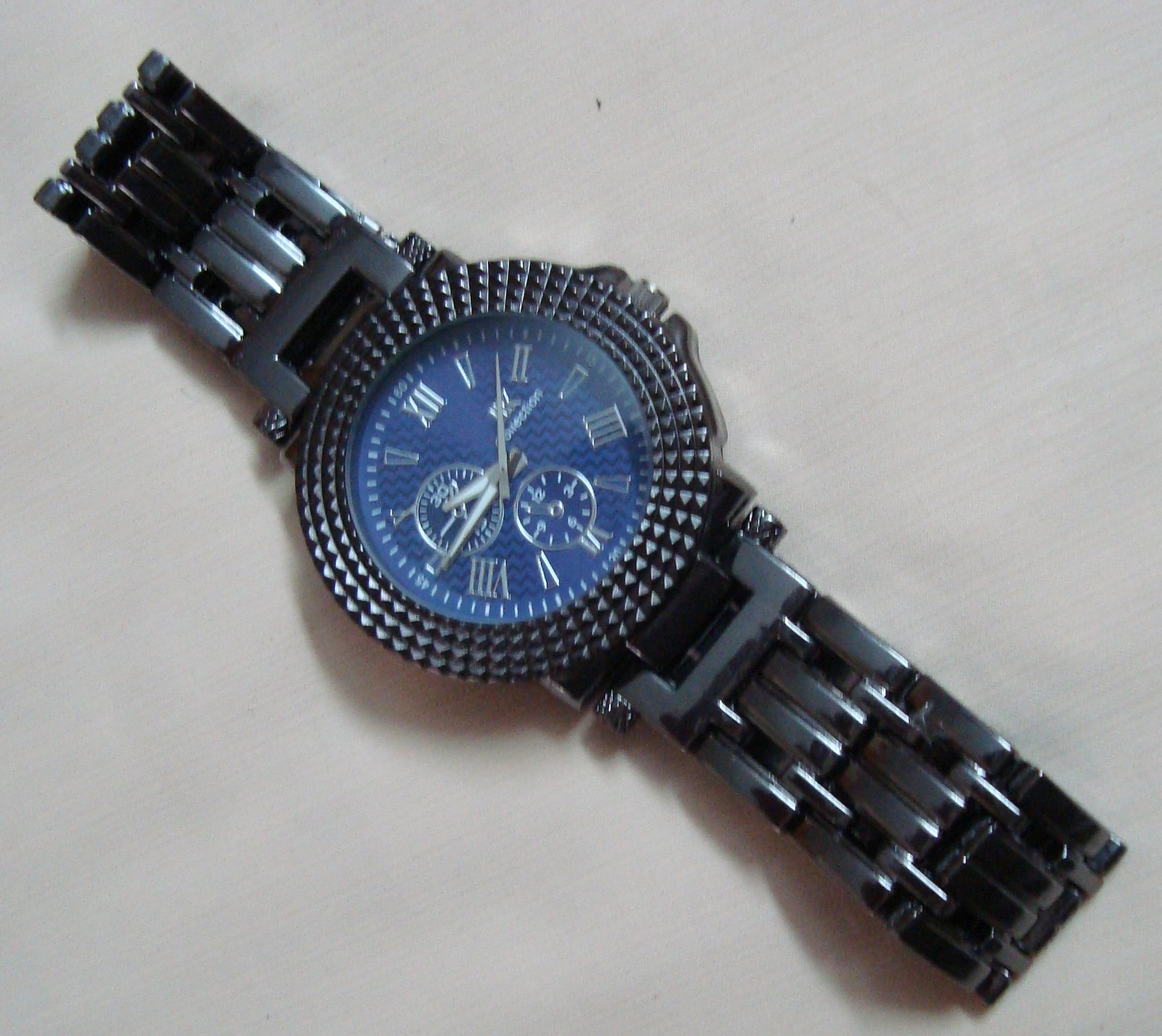In the photograph, there is a close-up, slightly blurry image of a men’s wristwatch diagonally positioned from the bottom right to the upper left of the frame, casting a shadow to its left. The watch rests on a light-colored countertop with a subtle striped pattern. The watch features a rough-textured, metallic black bezel framing a navy blue watch face. The face is adorned with silver Roman numerals indicating the hours from 1 to 12, along with silver-colored hour, minute, and second hands. The watch also contains two smaller dials at the 9 o'clock and 6 o'clock positions, possibly for setting different time zones or other functions. The time displayed on the watch is approximately 9:45, with the second hand located midway between the 1 and 2. Additionally, the watch includes an adjustment dial on the right side at the 3 o'clock position. The band of the watch is black, enhancing its sleek and sophisticated appearance.